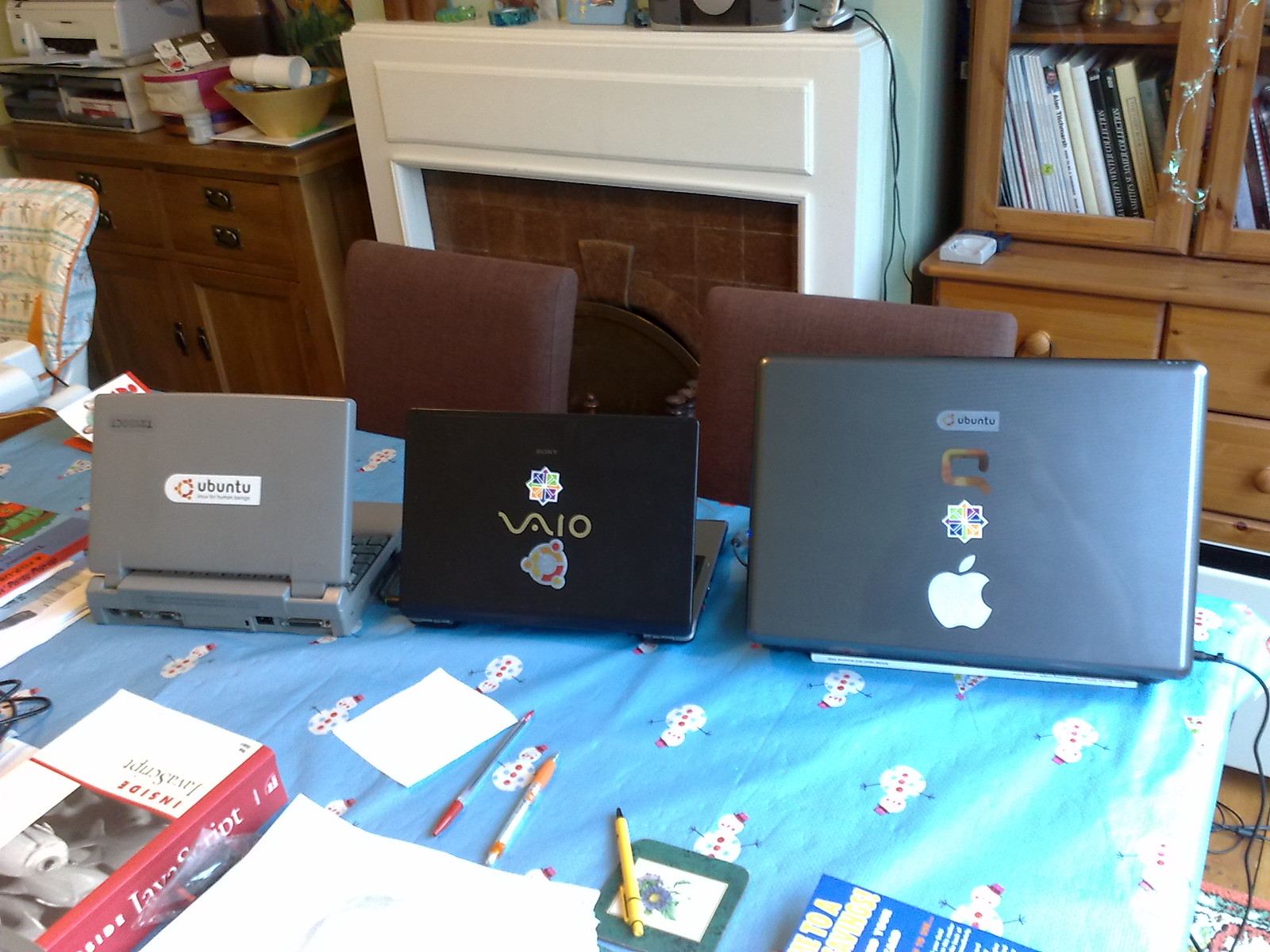This detailed image captures a cluttered home office or possibly a dining room transformed into a temporary workspace. The centerpiece is a rectangular table draped with a light blue tablecloth adorned with cheerful snowmen wearing red hats. On the tabletop, three open laptops face the camera. 

The laptop on the left is the largest and appears to be a vintage Apple MacBook, noting its silver color, recognizable Apple logo, and various stickers, including an Ubuntu sticker with black lettering on a white background, and colorful geometric and circular designs. 

The middle laptop is a black Sony VAIO. It also features multiple stickers, including a geometric pattern in yellow, green, and blue, and another with circles in yellow, orange, red, and white. 

The smallest laptop on the right is thick and chunky with a somewhat blurred brand identification but includes an Ubuntu sticker among others. 

The table is scattered with items: papers, pens of various colors (yellow, white and orange, clear glass with a red cap), and books, notably a thick JavaScript programming book. 

Surrounding the table are two brown chairs, and in the background, a cluttered room reveals an unlit brick fireplace with a white surround, a baby high chair, and shelves overflowing with books. The entire setting gives a sense of a busy, multipurpose space rich with detail and personal touches.